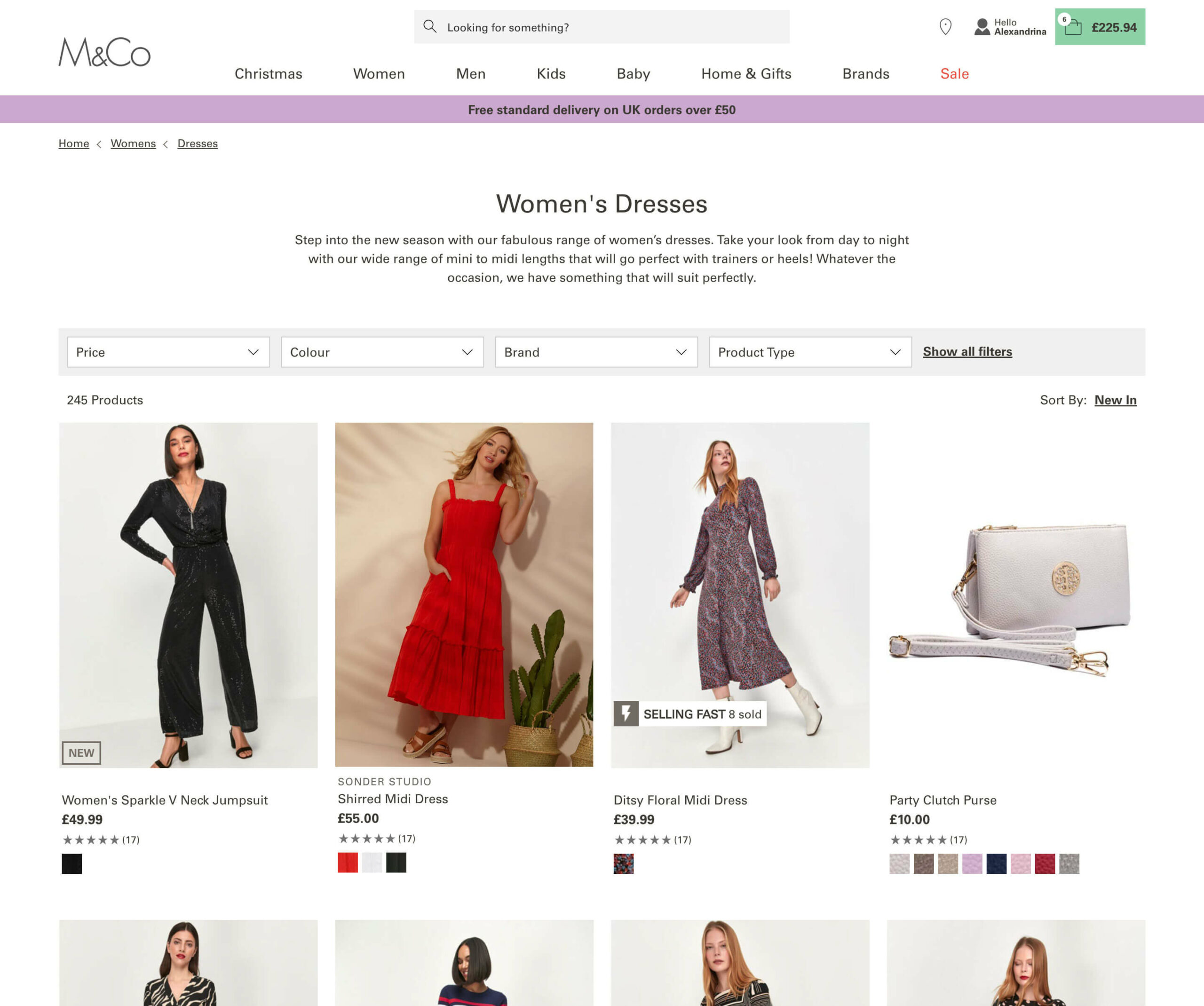This image, sourced from the MNCO website, features a clean white background. At the top center of the page, a search bar is prominently displayed with the placeholder text "Looking for something?". To its right, there are icons for user account management and a shopping cart, the latter indicating a total of £225.94 in selected items.

Below this header, there is a navigation menu, spanning from left to right, with tabs labeled: Christmas, Women, Men, Kids, Baby, Home, Gifts, Brands, and Sale. Beneath this navigation menu, a category section is visible on the left side, with labels for Home, Women's, and Dresses, the specific section captured in the screenshot. 

In this section, a banner announces "Free Standard Delivery on UK Orders Over £50". Below this banner, the category title "Women's Dresses" appears, showcasing a selection of items. The top row displays four distinct dress options modeled by women. However, it is notable that the top right item in the second row diverges as it features a clutch bag instead of a dress, distinct from the other items.